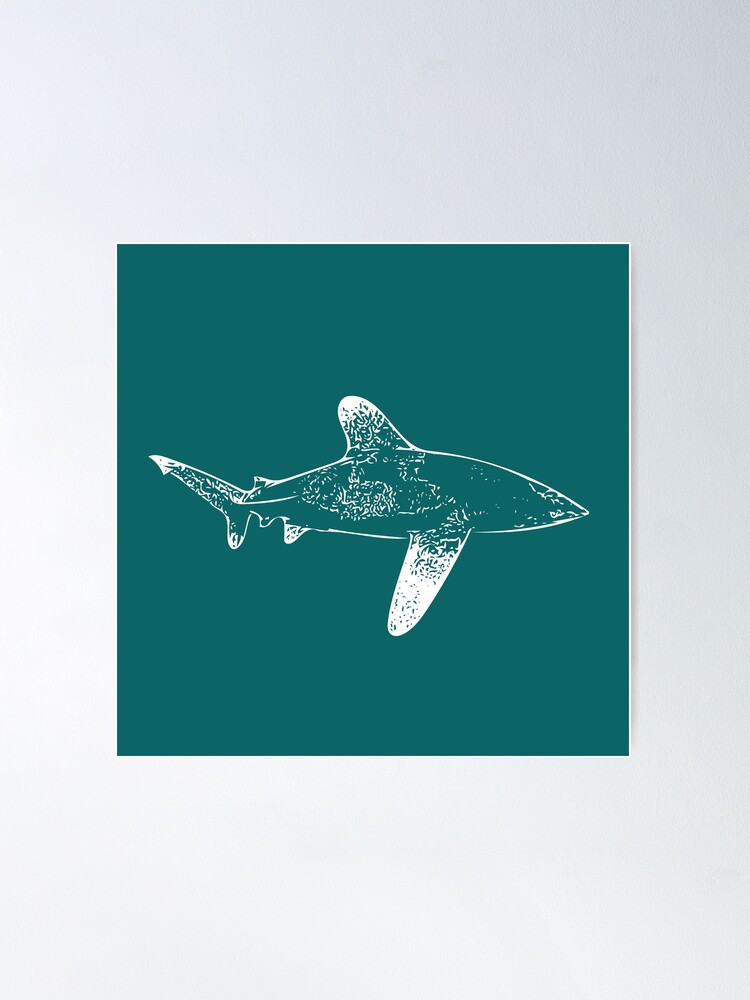The image showcases a piece of minimalist artwork characterized by its simplicity and limited color palette. Set against a very pale blue or light gray background, there is a central dark greenish-teal square that frames the focal illustration. Inside this square, a white outline of a shark is depicted, facing to the right. The shark illustration is minimalistic, with sparse details that include a series of fins—one long bottom fin, a shorter top fin, several tiny fins, and a long fin towards the upper back near the tail paired with a shorter one below. The white shark illustration appears hand-painted, with different splotches of white giving it a textured effect that allows the underlying teal color to peek through. This effect contributes to the depth and texture of the image, despite its overall minimalist aesthetic. The face of the shark is not well-defined, adhering to the minimalistic style, and emphasizing abstract simplicity.